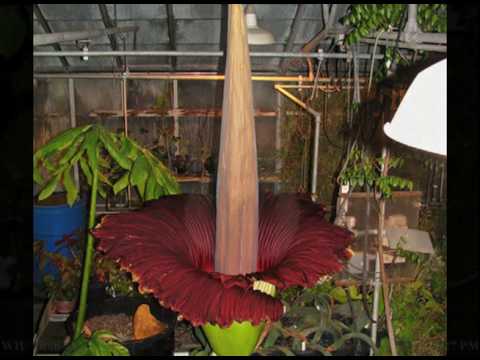This photo, meticulously bordered in black, captures an indoor greenhouse scene with an array of intricate details. Dominating the image's center is a strikingly deep red flower in full bloom. From its vibrant green base, a large light brown stamen extends upward, reaching beyond the frame. The setting, illuminated by late evening or nighttime light, features rusted, orangish-yellow metal posts forming the greenhouse structure, with glass panels partially visible at the top. Surrounding the central blossom are nondescript green stalks, adding to the lushness of the scene. Additional elements include a blue rain barrel on the lower left, a black pot slightly left of center, and a white lampshade peeping from the upper right. The overall ambiance hints at a well-maintained yet rustic indoor garden space, showcasing a variety of natural hues like green, red, brown, and gray against a backdrop of glass and metal.